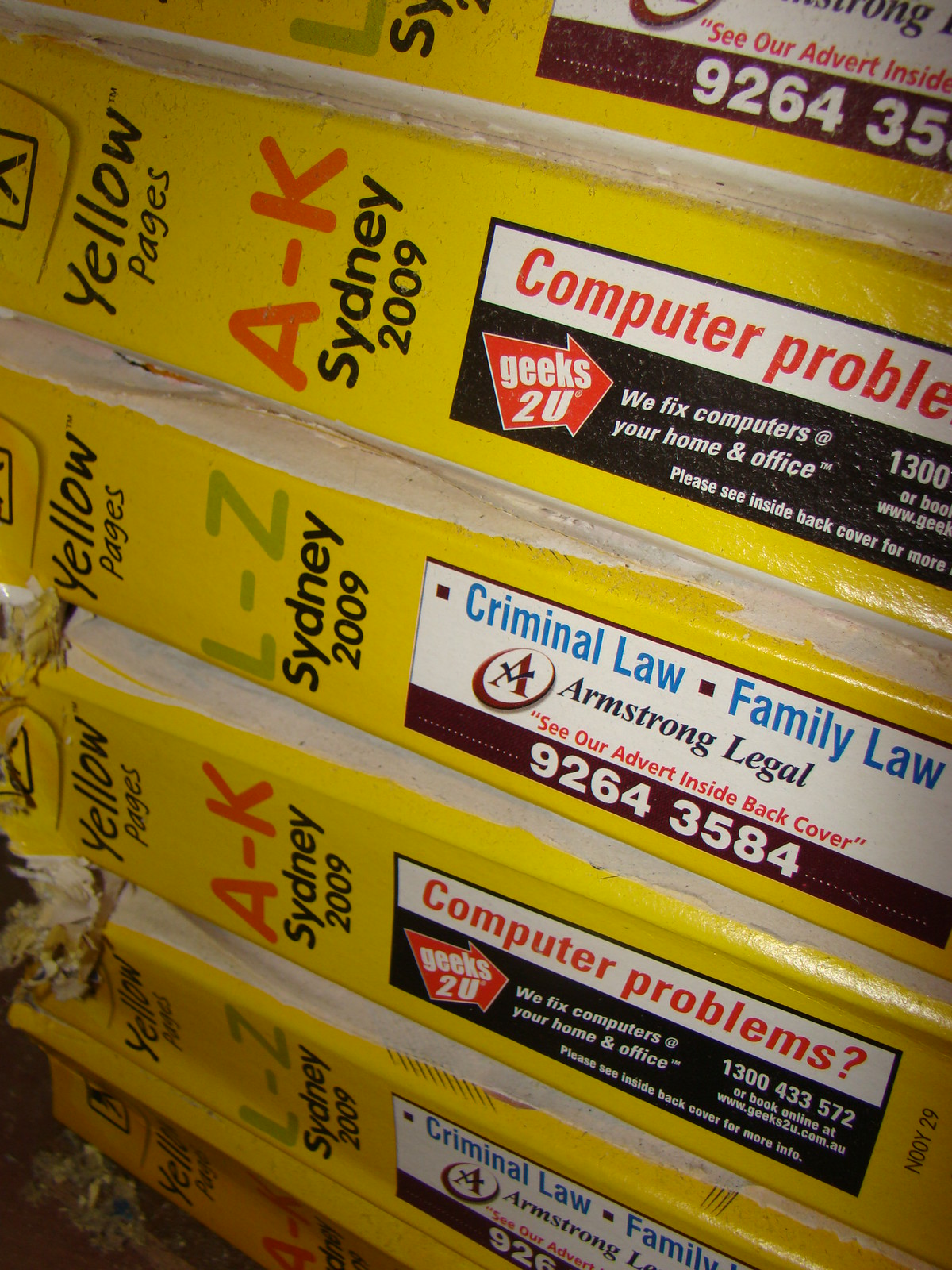The photograph, taken in portrait mode with flash, captures a stack of well-worn Sydney Yellow Pages from 2009, sorted in alphabetical order. The books are arranged alternately, with volumes labeled "A-K" and "L-Z" on their spines. Each spine features black font stating "Yellow Pages" and "Sydney 2009". The A-K volumes include an advertisement for computer repairs in a black box stating, "We fix computers your home and office," followed by a phone number. The L-Z volumes have an ad in a white box, highlighted in blue letters for "Criminal Law Family Law," and in red letters the firm "Armstrong Legal" with the note "see our advert inside back cover." The condition of the books shows significant wear and tear, especially on the spines, with the bottom L-Z volume displaying crinkled and ruffled edges, indicating its age and use.